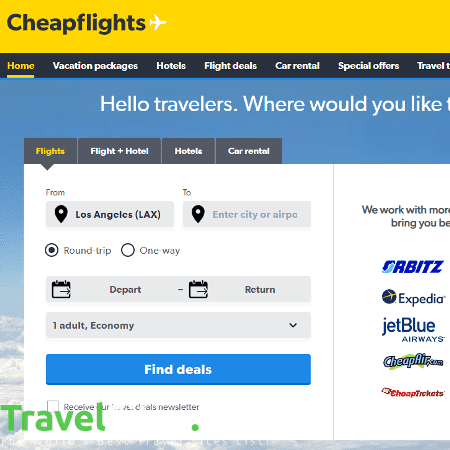A detailed screenshot from a computer displays a partially completed search form for cheap flights on a travel website. At the top, a yellow banner with the text "Cheap Flights" in black is prominently featured. Below this header, the "Home" tab is highlighted in yellow, indicating it has been selected, with an underline accentuating its status. 

In the next section, a blue bar greets with the phrase "Hello travelers, where would you like..." followed by a cutoff, suggesting a welcoming message that continues beyond the visible area. Another yellow-highlighted tab indicates the "Flights" section has been selected. The search form shows inputs labeled "From" and "To," where the user has entered "Los Angeles (LAX)" in the "From" field, but left the "To" field blank. The user has selected a "Round Trip" option and specified travel details as "1 Adult, Economy."

Below these inputs, a prominent blue button labeled "Find Deals" is ready for activation once all required fields are filled out. In the bottom left corner of the screenshot, the word "Travel" appears in green. Meanwhile, on the right side of the screen, a sidebar beginning with "We work with" is visible, though truncated, displaying logos of partnering companies such as Expedia and JetBlue Airways, among others.